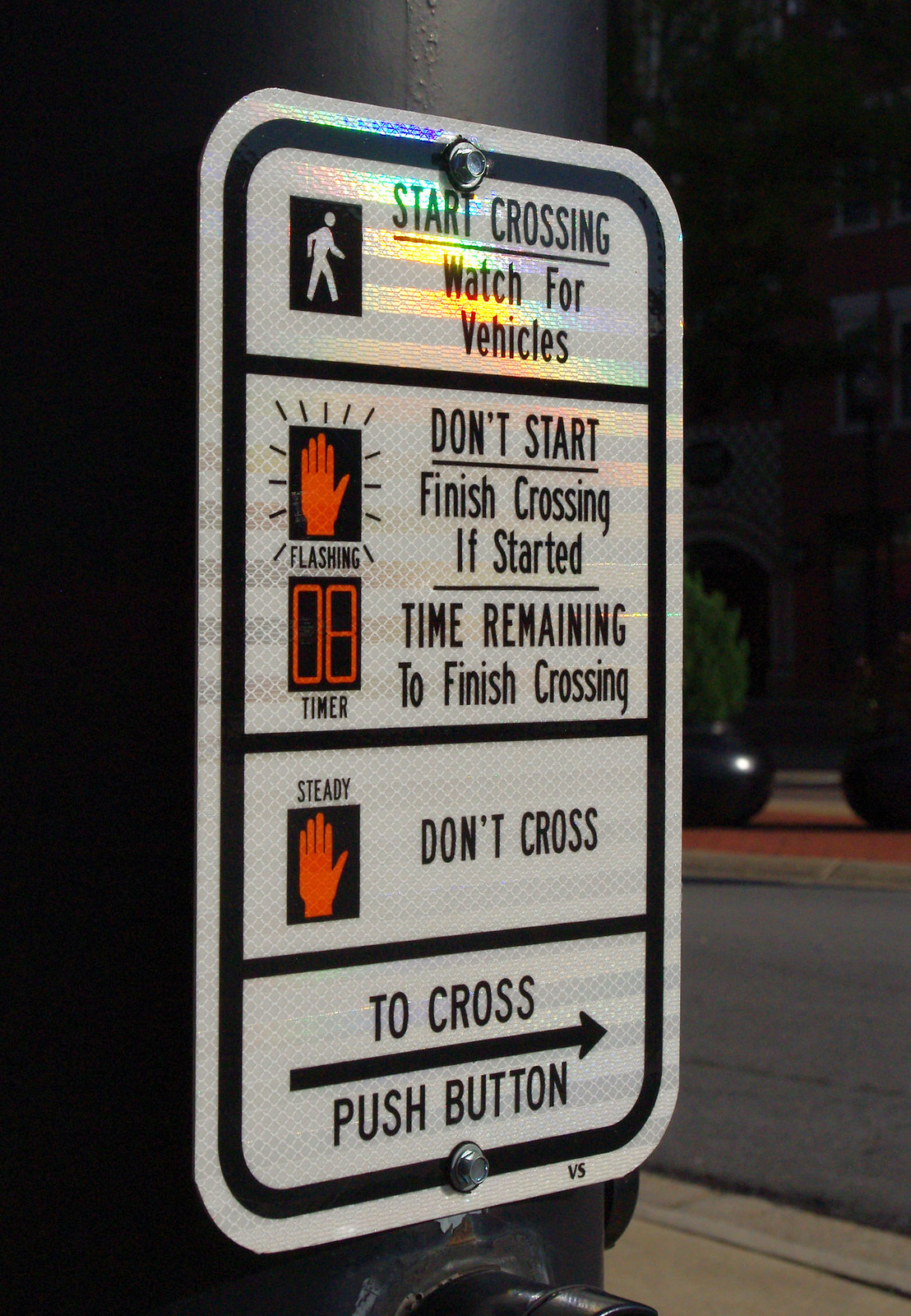The image features a white, four-segment pedestrian crossing sign mounted on a black object, secured by screws at the top center and bottom center. The sign is photographed at an angle, emphasizing its detailed instructions and icons. 

In the top segment, there is an icon of a person walking, accompanied by the text "Start Crossing Watch for Vehicles" in black font. The second, larger segment includes two icons: one with an orange hand labeled "Flashing" and another showing "08" in orange letters, alongside the text "Timer." To the right, it states, "Don't Start Finish Crossing if Started Time Remaining to Finish Crossing." The third segment features an orange hand labeled "Steady," with the instruction "Don't Cross" beside it. The bottom segment directs pedestrians, "To Cross Push Button," accompanied by an arrow and a clear metal button to press.

The setting appears to be outdoor, potentially nighttime, suggested by the lighting conditions and the faint presence of a car and street light in the background. The image captures a crucial street element focused on pedestrian safety, providing clear and detailed crossing instructions.